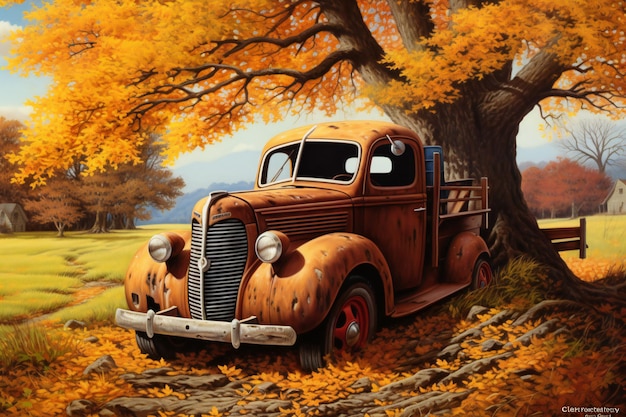The image is a digitally-generated depiction, mimicking a rustic country painting, set in a vibrant autumnal scene. Central to the image is a 1920s pickup truck, positioned diagonally with its front facing slightly towards the left. The truck, a rusted orange hue, is heavily pitted and dented, particularly around the fender wheels and wheel wells, and it features striking red rims. The tires are either sunk into the ground or buried under a thick layer of fallen autumn leaves. Notably, its side mirrors are mounted on the roof, unlike the usual placement near the windshield. 

This vintage vehicle is parked under a sprawling oak tree, which is ablaze with brilliant orange foliage. Leaves from this tree cascade down, carpeting the roots and rocky ground beneath it. To the left of the scene, light green grass extends towards the horizon, punctuated by the presence of more autumn-colored trees and a distant forest. In the background, slightly to the right and partially obscured by the tree, a white farmhouse with a peaked roof is visible, adding to the charm of the countryside setting. Further enhancing the landscape are grassy fields and distant mountains, completing this picturesque, digitally-crafted autumn scene. In the bed of the truck lies a mysterious blue object, adding a touch of intrigue to the rustic atmosphere. The bottom right corner of the image contains an indistinct signature, possibly referencing a website, factory.com.